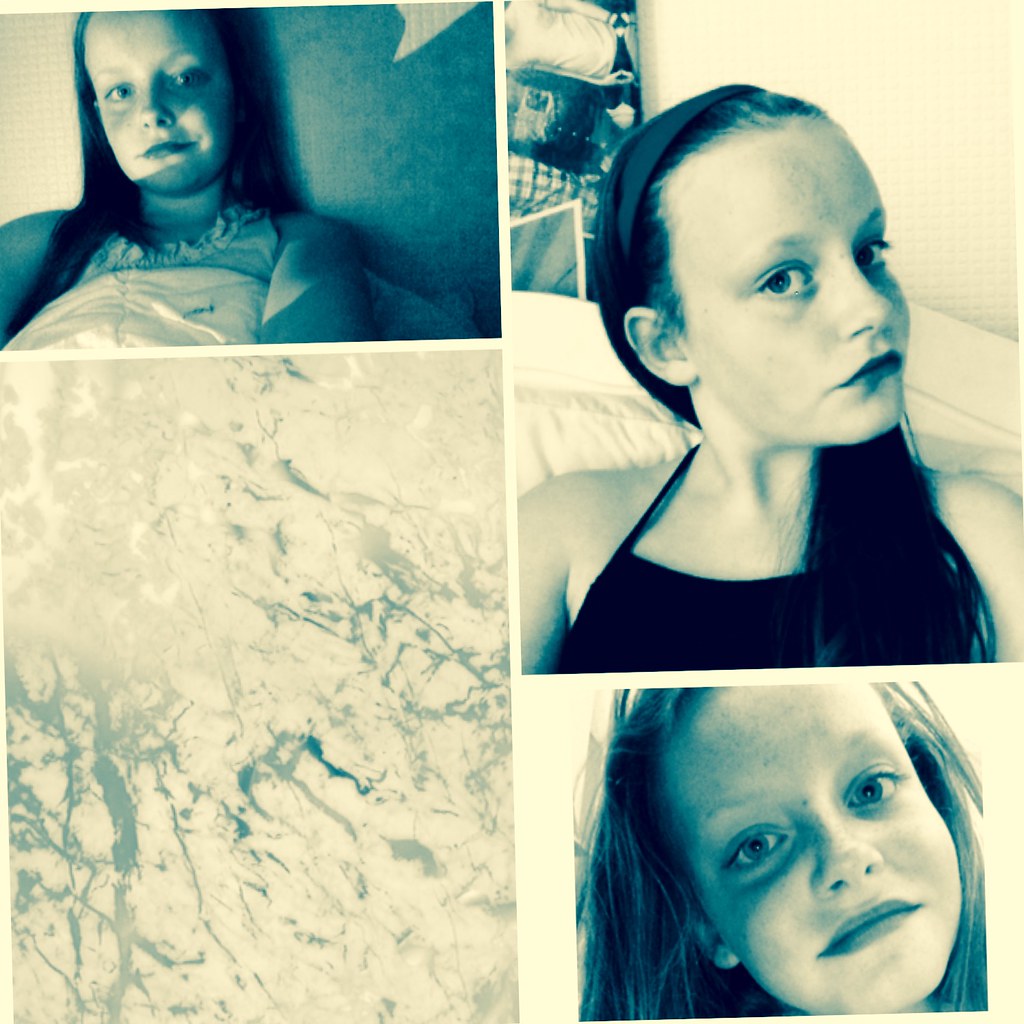The image features a detailed collage of a young adolescent girl, captured in a series of four distinct, black-and-white tinted photographs with a dark bluish overlay. The top left frame shows the girl reclining, perhaps against a headboard in a dimly-lit room, with her long black hair pushed back and a blanket covering her partially. Adjacent to it, in the top right frame, the girl is seated with her hair over one shoulder, wearing a black tank top and a headband that pulls her hair back, against a white background, seeming to take a selfie. The bottom left frame diverges from the rest, portraying an abstract scene reminiscent of ice on a window, with white and clear lines intersecting. Finally, the bottom right frame offers a close-up of the girl's face, highlighting her youthful features and direct gaze at the camera. This candid and intimate collage appears to have been crafted by the girl herself, possibly as a reflection of her everyday moments or intended for sharing on social media. The absence of text and the varying settings, predominantly indoors, lend an air of personal and spontaneous expression to the compilation.